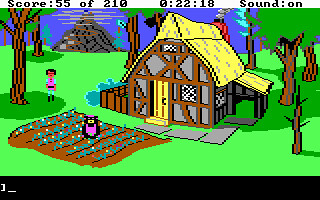The image appears to be a screenshot from a video game. At the top, there is a white strip with black text that reads "Score: 55 of 210." The interface indicates that the sound is on, with a timer displaying 0:22:18. The focal point is a barn, featuring a yellow roof accented with subtle gray lines. The front of the barn is gray, supported by brown wooden beams, and includes a yellow door and a black-and-white window. Surrounding the barn is a lush expanse of green grass, punctuated by a small garden. In the garden, a small, purple owl with black edges can be seen. The background is filled with numerous trees covered in green leaves. Among these trees is a little girl dressed in purple, standing near what appears to be a large pile of wood.